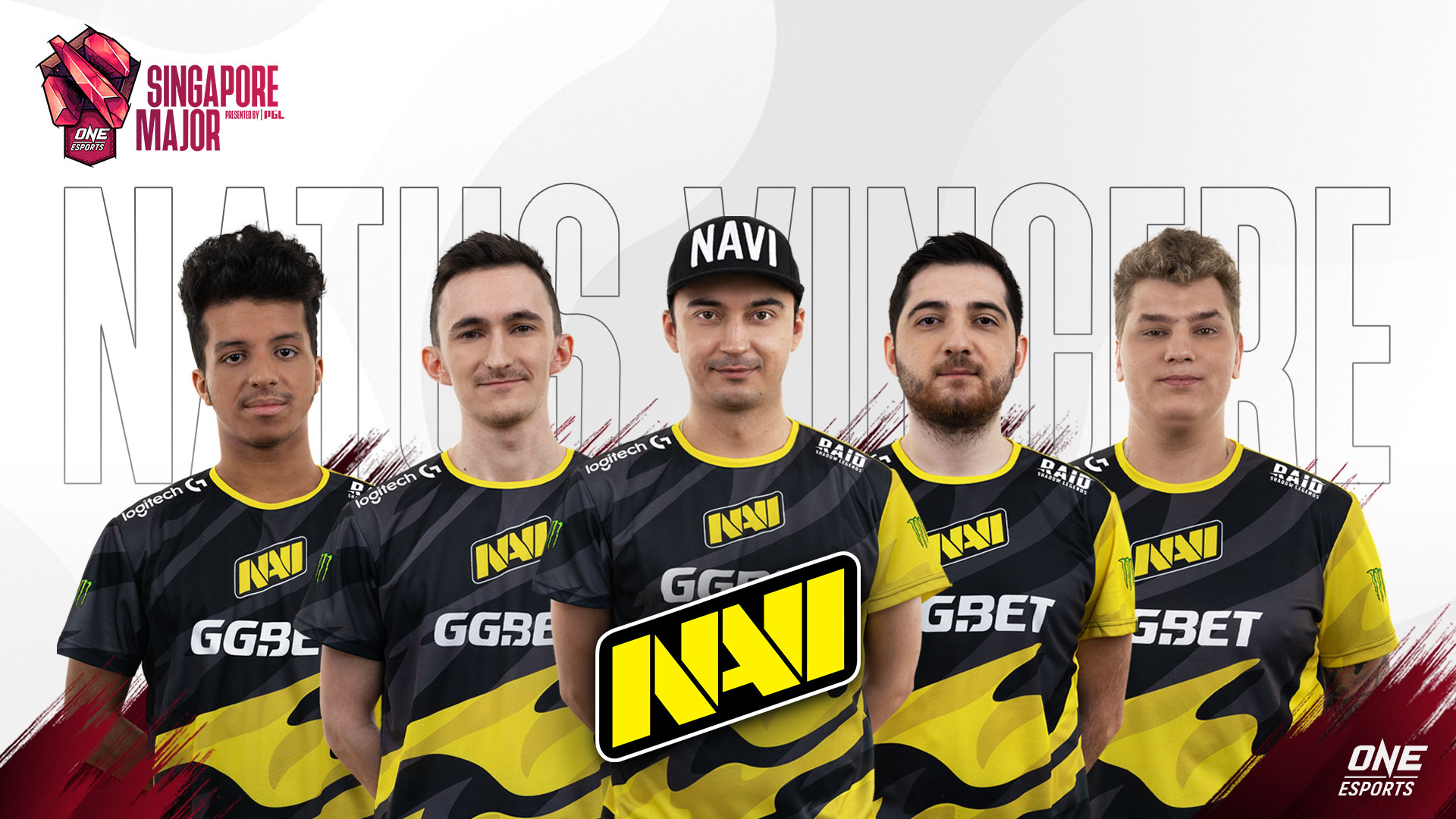The photograph depicts six young men standing in the foreground, all wearing matching short-sleeved black jerseys with yellow trim. The jerseys feature various texts including "NAVI" prominently displayed across the chest in yellow letters, with additional text like "GG.BET" in the lower right corner and "One Esports" also visible. The man in the middle is distinguished by a black baseball cap bearing the "NAVI" logo in white letters. The background of the image shows partially obscured lettering, making it difficult to read. In the top left corner of the image, a red stylized logo along with the text "Singapore Major presented by PGL" is clearly visible. The bottom of the image also contains text, but it is hidden behind the players. The photograph itself is wider than it is tall, and the overall setup suggests that these men are part of a sports team, likely representing Singapore in this major event.